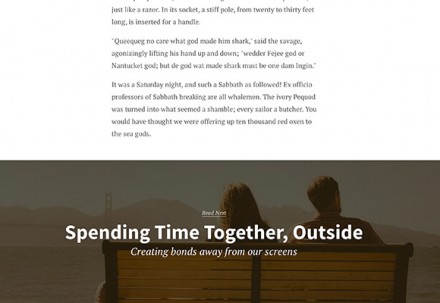**Detailed Caption:**

This image, titled "Spending Time Together Outside," is split into two primary sections. The upper section has a plain white background with centered black text arranged in three paragraphs. The first paragraph states: "Just like a razor in its socket, a stiff pole from 20 to 30 feet long is inserted for a handle." The second paragraph reads: "Quiggerig, no care what god made him shark, said the savage, agonizingly lifting his hand up and down. Wetter Fiji god or Nantucket god, but de god, we at bed shark, but made damn furriga." The third paragraph describes a scene: "It was a Saturday night and such sabbath as followed. Ex officio professors of sabbath breaking are off, whale men. The ivory pickad was turned into what seemed a shamble, every sailor a butcher. You would have thought we were offering up 10,000 red oxes to the sea gods."

Beneath the text, a long rectangular image portrays a serene outdoor scene. In the foreground, a Caucasian man and woman are seated side by side on a wooden bench crafted from light blonde wood with a black frame. They are engaging in conversation or simply enjoying each other’s company. Behind them, the scenery expands to reveal three majestic mountains, a bridge, and a bay opening into the ocean, creating a picturesque and tranquil backdrop.